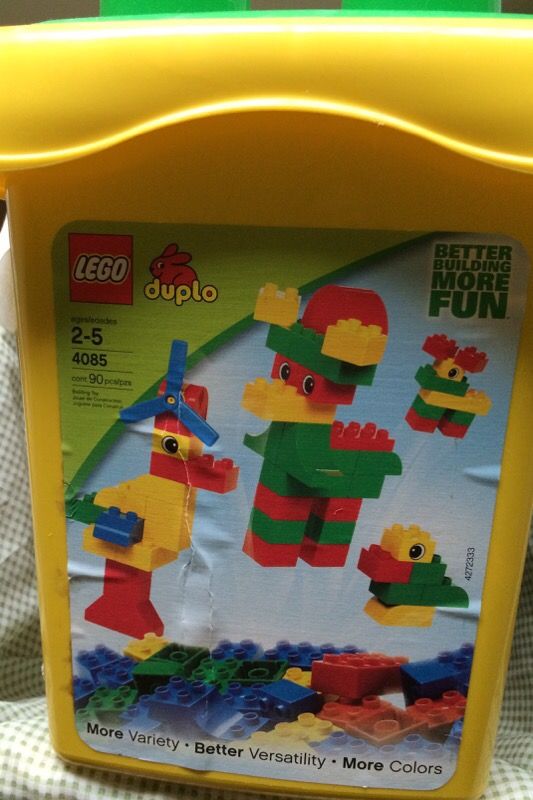The image showcases a Lego Duplo building block toy set contained in a square yellow bucket with a matching yellow lid. The front of the bucket features a large rectangular sticker, which illustrates multiple buildable animals including a duck, horse, moose, and a small bird, alongside a pile of colorful blocks. The sticker's top left corner has a green banner displaying a red square with white text that reads "Lego," along with a red rabbit above the yellow word "Duplo." The top right of the label, in green text, promotes "Better building, more fun." The text also notes the set is suitable for ages 2-5 and includes 90 pieces. The bucket is placed on a white and green checkered sheet, suggesting a kid-friendly environment, possibly a playroom. The bright colors of the blocks—red, yellow, green, blue, and white—are prominently featured, enhancing the visual appeal and emphasizing the variety and versatility of the set.